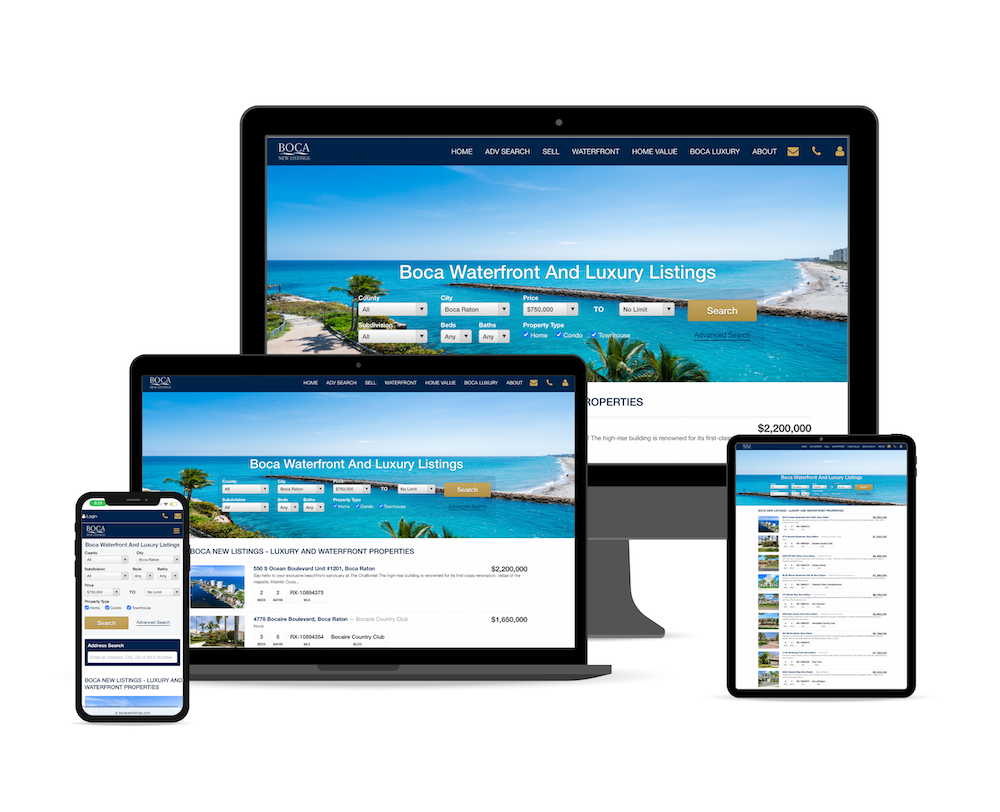The image displays multiple devices—a computer monitor, a laptop with its screen open, a tablet, and a smartphone—all showcasing the same website, "Boca Waterfront and Luxury Listings." Each device's screen is clearly visible and the website is uniformly displayed across all of them, highlighting its responsive design. The website's homepage is prominently featured with a visually appealing image of a scenic waterfront. This image includes a beach with palm trees, a dock extending into a lagoon area, and a view of the expansive main waterway. 

At the top of each screen, the website’s navigation tabs are visible, including options such as Home, Advanced Search, Waterfront, Home Value, Boca Library, and About. Additionally, there are icons for email, phone, and user accounts. Notably, the smartphone does not display the aforementioned waterfront image but still shows the consistent layout of the website. This showcases the versatility and adaptability of the Boca Waterfront and Luxury Listings website across various devices.